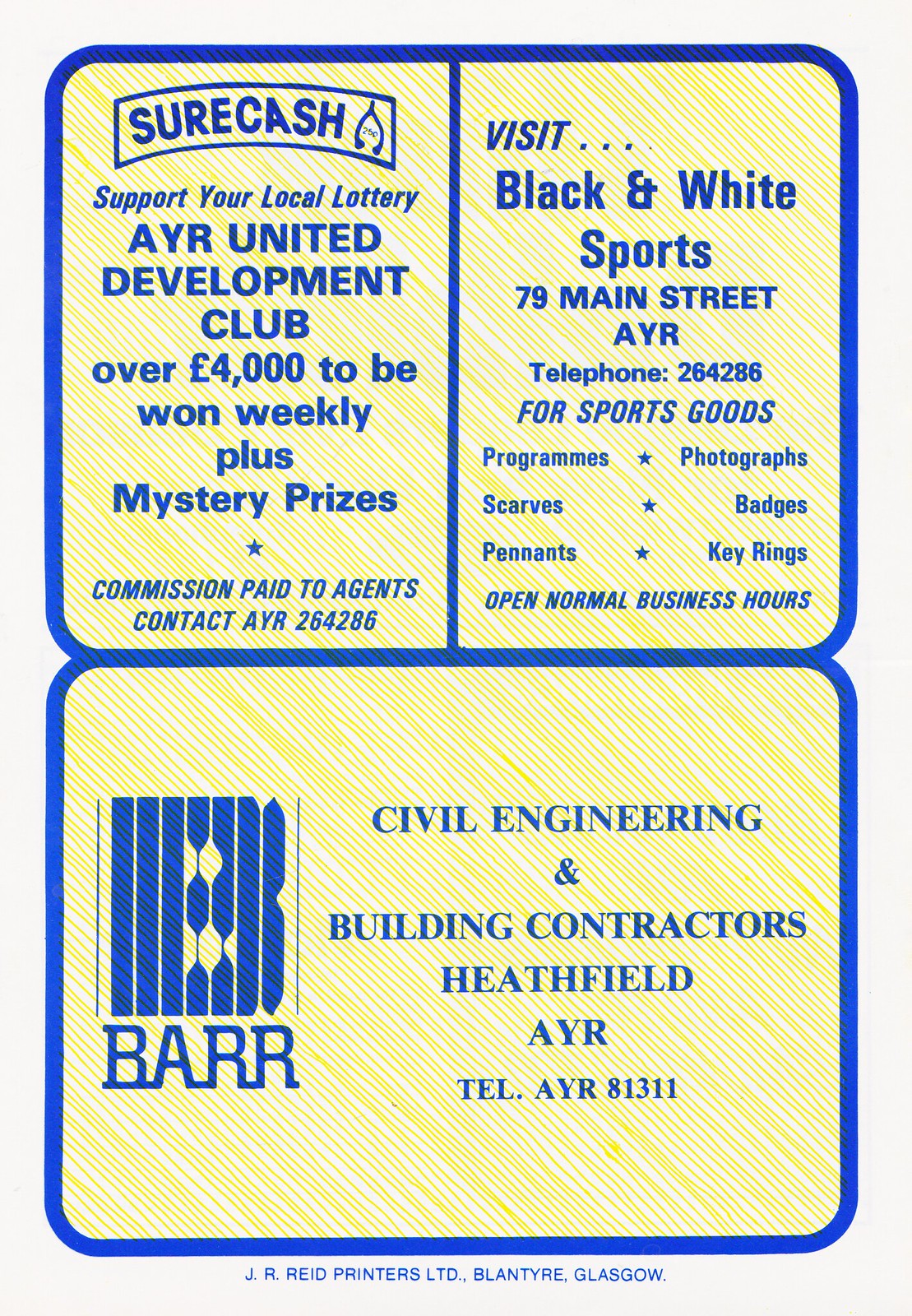A vintage advertisement poster divided into three sections with a consistent yellow striped background and blue borders. The top half features two sections: the left side advertises "Sure Cash" for the AYR United Development Club, highlighting weekly winnings of over £4,000 plus mystery prizes. Supporting local lottery, it's accompanied by a contact number (AYR 264-286). On the right, another section promotes "Visit Black and White Sports" located at 79 Main Street, AYR, offering sporting goods like programs, scarves, pennants, photographs, badges, and key rings. This section notes the store's address and contact details, emphasizing "Open Normal Business Hours." The bottom half of the poster, in a larger, banner-like section, advertises a civil engineering and building contractor named "BAR" with a notable logo of vertical stripes and the text "Civil Engineering and Building Contractors, Heathfield, AYR." The contact number provided is AYR 81311. Additionally, small print outside the blue border at the bottom credits "J.R. Reed, Printers Ltd., Land Tire, Glasgow."